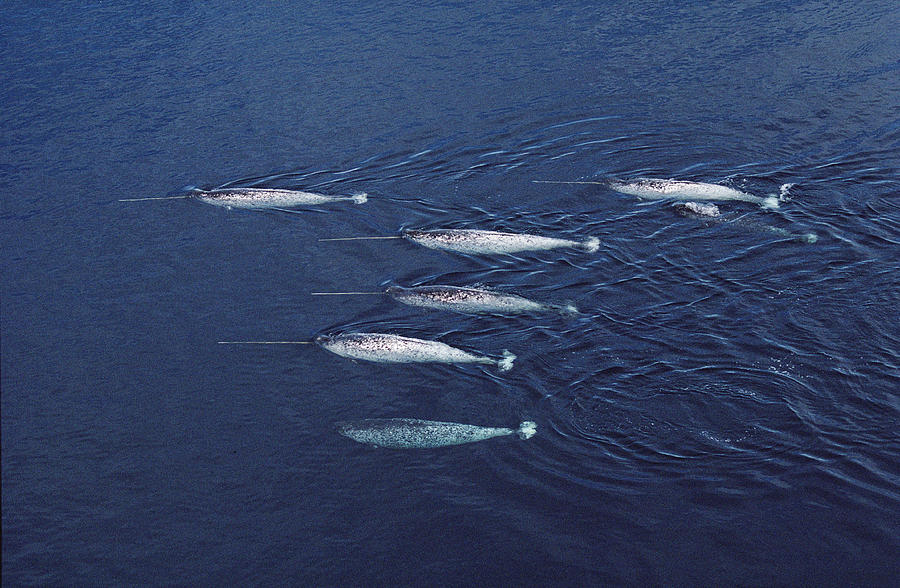This horizontal rectangular image showcases a vibrant ocean scene featuring six unique, large, and narrow fish swimming near the surface of deep, dark blue water. The fish are all moving in the same direction, towards the left side of the image. Notably, five of the fish have long, needle-like appendages extending from the tops of their heads, resembling silver poles aimed to the left. The fish exhibit a white and speckled bluish coloration, skimming gracefully along the water's surface, creating subtle ripples. One of the fish, positioned at the bottom, lacks this distinctive appendage, adding to the intriguing composition of the scene.